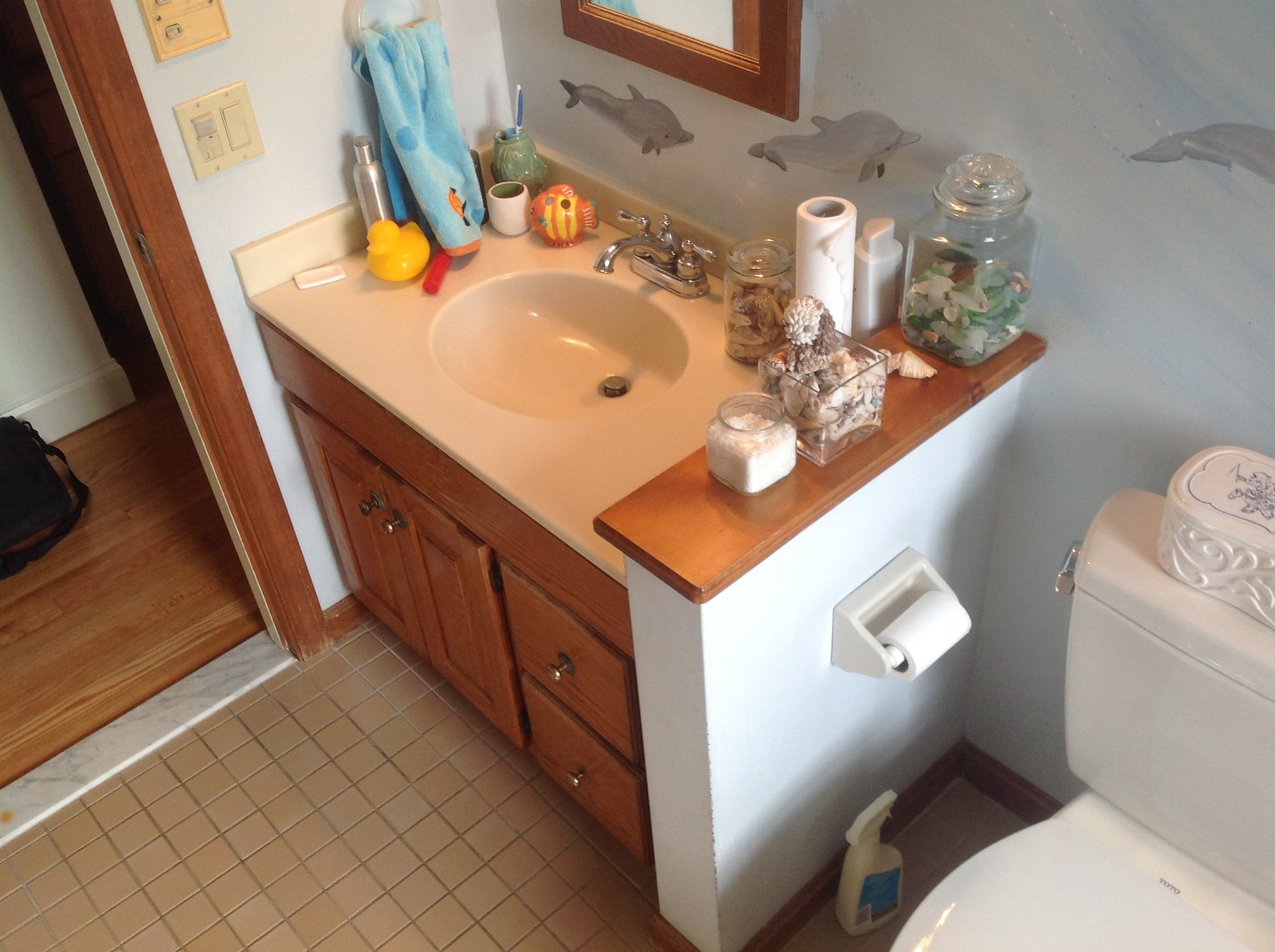The image is a color photograph taken from an unusual high angle looking down into a bathroom. The entry door features a marble threshold, separating the bathroom from the adjacent hallway with its hardwood floor and white walls. Just outside the bathroom, a dark-colored handbag or suitcase is visible in the hallway.

Inside the bathroom, the floor is covered with small square tiles. The vanity is an aged medium oak piece matching the trim around the door. Two ivory-colored rocker light switches are installed by the entrance, above which is an old intercom system reminiscent of the 1970s. The single-sink vanity has a formed composite top, giving it a simple, possibly child-friendly appearance. A light blue towel with dark blue polka dots is hanging on a ring on the wall, featuring a playful design. A yellow rubber duck sits on the counter beside a fish-shaped toothbrush holder and another caddy or holder.

A framed mirror above the sink matches the wood tones of the door and vanity. The chrome faucet includes hot and cold handles. Various glass jars adorn the countertop, including one filled with seashells, suggesting a beach-themed decor rather than a purely child's bathroom. The walls are painted blue with hand-painted waves and dolphins, giving the space a whimsical touch. One dolphin is swimming above the sink, another higher up, and one more above the toilet.

A low dividing wall separates the sink from the toilet, topped with a brown wooden counter-like surface. This area holds a square stopper jar of sea glass, more seashells, a jar possibly containing cotton balls, and another square container with additional seashells. A white toilet paper holder is mounted to the wall, while the toilet itself has an ornate box on its tank lid. A spray bottle rests on the floor next to the toilet, completing the scene.